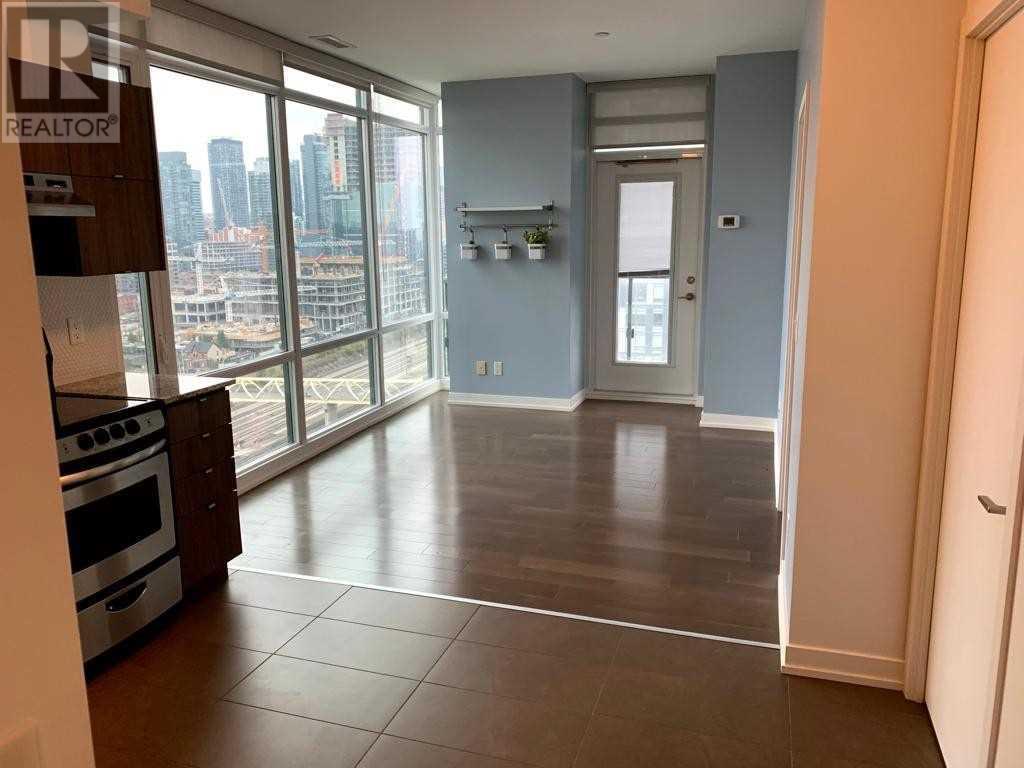This image, sourced from a Realtor website, offers a view from the kitchen into an adjacent room within an apartment. The image includes a watermark in the upper left corner, featuring a square with a central "R" and a white border labeled "Realtor" at the bottom. 

The kitchen is equipped with a brown tile floor and a stainless steel cooktop stovetop with four burners, controlled by dials located on the oven's front panel. The kitchen cabinetry is a striking dark brown wood adorned with brass pulls, complemented by a brown granite countertop.

The adjacent room, which appears to serve as a small living area, showcases dark, shiny wood flooring. The left wall is entirely composed of floor-to-ceiling windows, offering a panoramic view of distant urban skyscrapers. The far wall is painted light gray and features a clothes hanger alongside a doorway at its center, which leads out to a balcony. This doorway is white and includes a large rectangular window at its center, coupled with a screen and a transom window above it.

Lastly, the right wall in this living area has a light cream color and houses a door with a metal pull handle. Additionally, a thermostat is mounted on the gray wall, to the right of the doorway leading to the balcony.